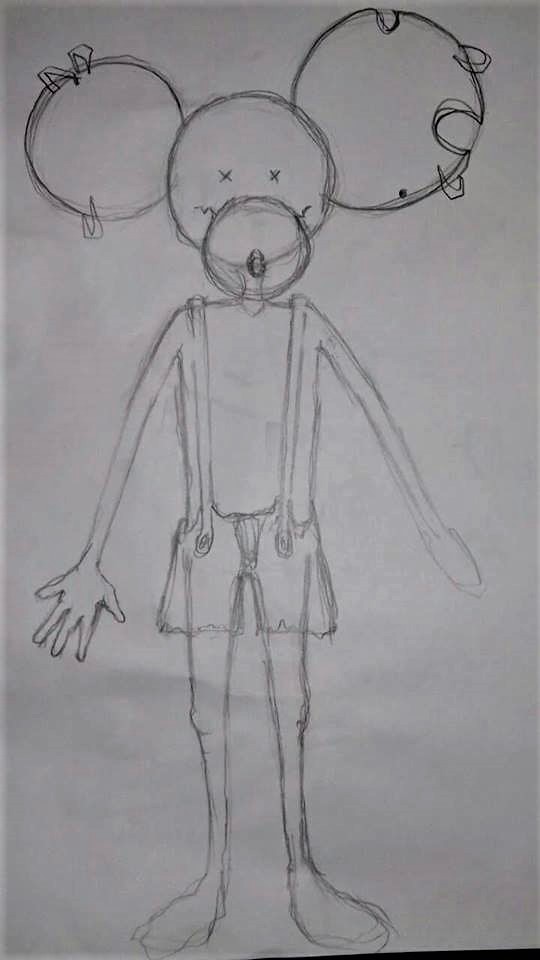This image depicts a sinister and unsettling version of Mickey Mouse. The character is dressed in a traditional outfit, consisting of a jumper attached to knee-length shorts. Unusually, Mickey has five fingers on his right hand, while his left arm ends abruptly at the wrist, devoid of any fingers. His ears are notably adorned with several piercings, especially on the right ear, while the left ear has both piercings and distinctive cutouts. His eyes are represented by simple X marks, adding to the eerie appearance. Complementing this are his crooked, squiggly-lined smile and a nose resembling an oblong button. His legs, which appear to lack toes, suggest he is not wearing shoes. The entire illustration is sketched with pencil on what appears to be a moderately crumpled piece of paper, enhancing the overall disturbing vibe of the artwork.